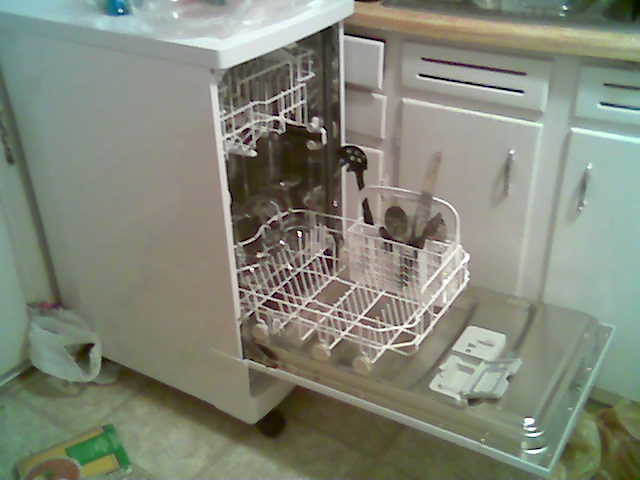This photograph captures a detailed view of a somewhat cluttered kitchen centered around a unique, portable dishwasher. Unlike a typical built-in model, this exceptionally narrow and wheeled dishwasher sits directly in front of the kitchen sink, obscuring access to the underlying cabinets and drawers. The dishwasher’s door is open, revealing the bottom rack pulled out with a few kitchen utensils such as a large knife and a black plastic spaghetti strainer placed in the silverware basket. The interior of the dishwasher features stainless steel and white racks. The countertop above is beige and cluttered with a couple of plates, hinting at a busy kitchen. The surrounding area shows white cabinets with plain silver hardware, and a red and black stripe detail on the top right drawers. The floor is covered in yellowish-beige tile squares, some relatively wide, possibly around nine or ten inches each, with a plastic grocery bag and a food package visible on the floor near the dishwasher.